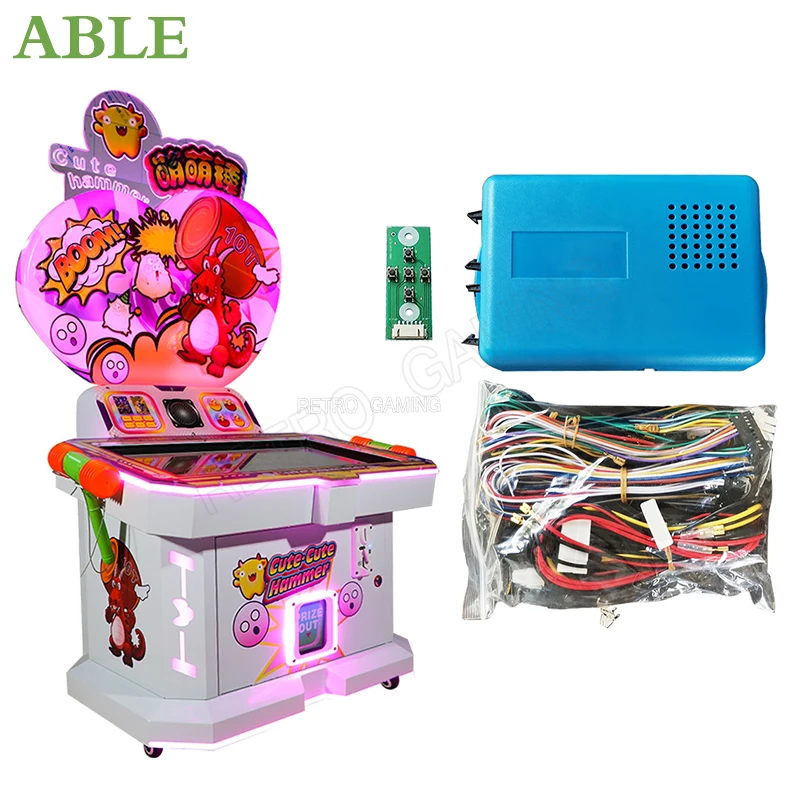The image features a life-sized or potentially miniature arcade game titled "Cute Cute Hammer," characterized by vibrant and playful colors including reds, pinks, purples, and greens. Situated on the left side, the arcade machine includes cartoon characters such as little pink balls with faces, yellow figures with faces, and pink dragons wielding hammers. The top of the machine has a touch screen display, and there's a backward sign that reads "boom." The top left corner of the image displays "Able" in green letters. To the right of the arcade game is a blue plastic case with ventilation holes, likely containing a battery pack, accompanied by a mini circuit board or motherboard. Below this blue case is a bag containing various colored cords, neatly arranged in hues like red, orange, yellow, and white. Centrally located, there are letters spelling out "Astro Gaming," though additional details are harder to discern.